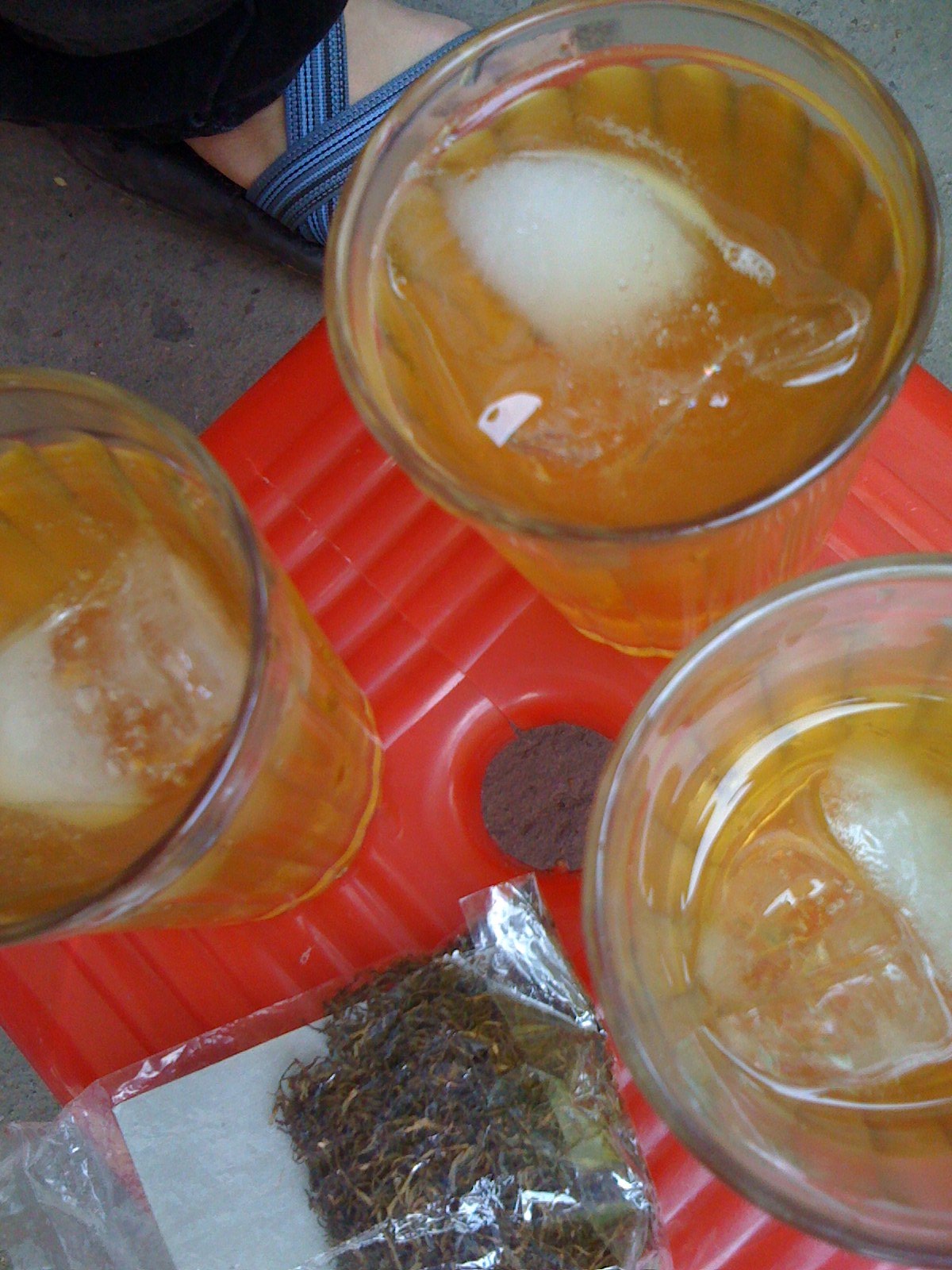This aerial view depicts a vividly detailed scene centered around a square, red textured serving tray. Three transparent glass tumblers, each filled to the brim with a white-yellow liquid resembling iced tea or light beer, sit prominently on the tray. Floating in each tumbler is a large, clear ice cube, notable for its shiny appearance and white center. The tray features a circular hole in its center. Adjacent to the tumblers, in the bottom left corner of the tray, rests a clear cellophane envelope containing a stringy, greenish-brown substance, possibly tea leaves or a similar material. In the background, the upper left-hand corner reveals a light-skinned foot clad in light blue and dark blue strappy sandals with black soles, hinting at the presence of a nearby individual.